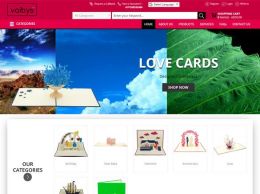This is a screenshot of an e-commerce website featuring a compact yet vibrant interface. The top header, adorned with a maroon-pinkish red background, houses the site’s logo, navigation menu, and search bar. Beneath this, a prominent header image displays a collage of various pictures, overlaid with large white text that reads "Love Cards." Directly below, the section titled "Our Categories" showcases a series of product photos that appear to be intricate, possibly pop-up cards. Despite the image’s pixelation and small size, the products seem elaborate and artistically designed. Positioned toward the center-right of the header image is a dark gray button with white text that invites visitors to "Shop Now," encouraging immediate engagement with the site’s offerings.